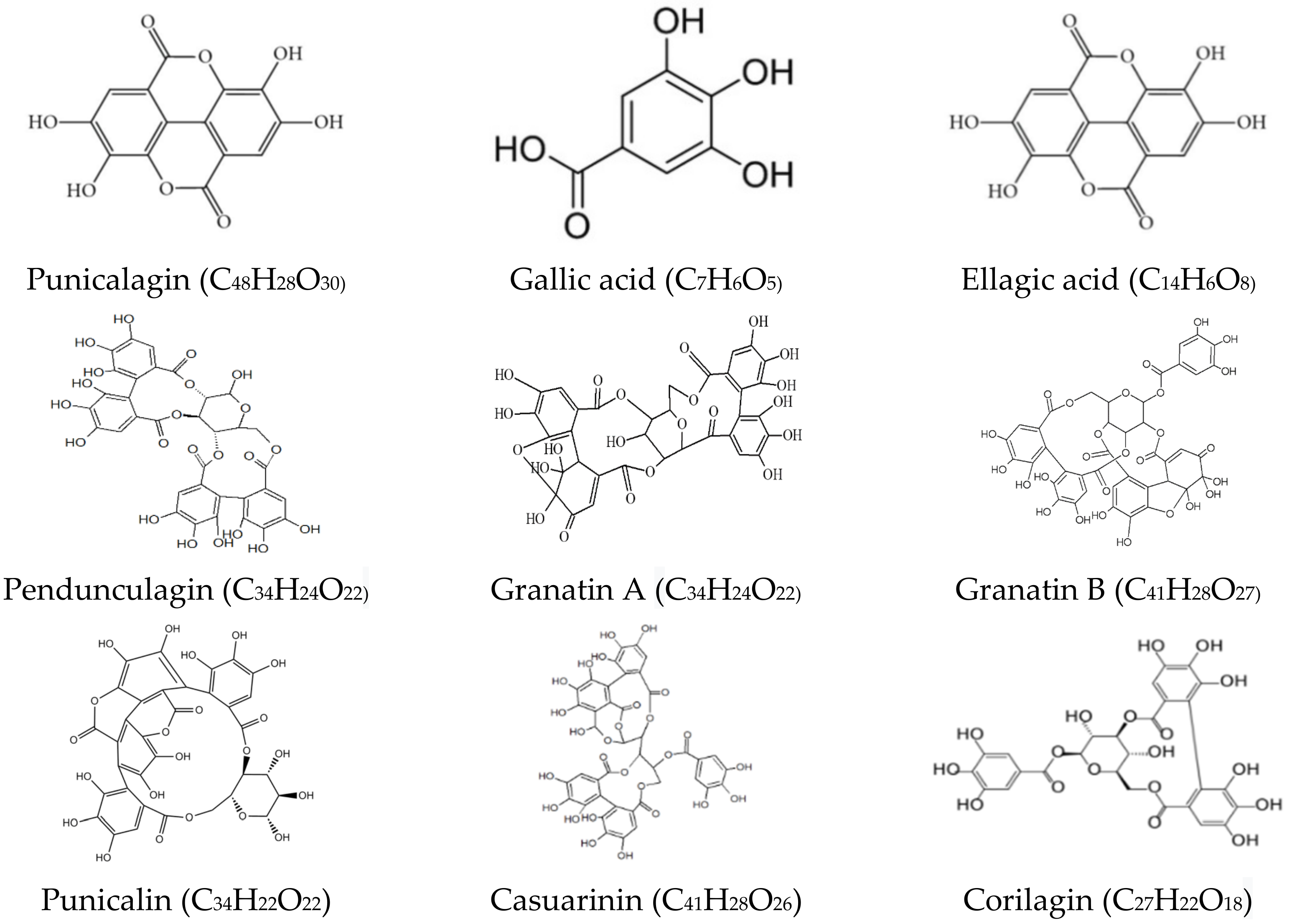The image depicts a scientific diagram with black text and molecular structures sketched in black on a white background. It shows nine different molecules presented in a three-by-three grid. Each molecule's name and scientific nomenclature are listed beneath their corresponding structure. The molecules are Punicalagin, Gallic Acid, Ellagic Acid, Pedunculagin, Granatin A, Granatin B, Punicalin, Casuarinin, and Corilagin. The molecular structures are detailed, depicting clusters of six-sided figures with various offshoots bearing O (oxygen) and OH (hydroxyl) groups.